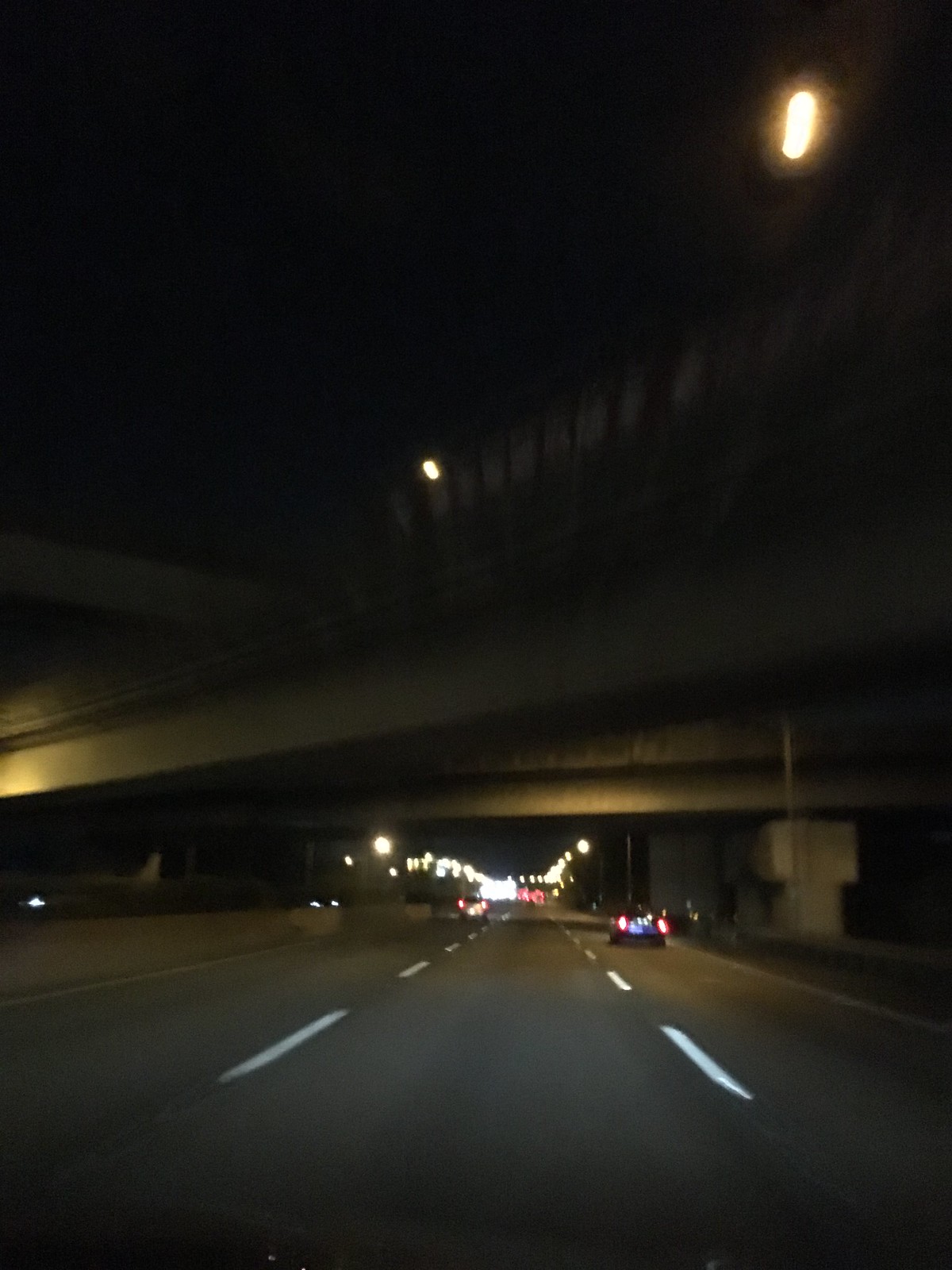This digital photograph captures a night-time scene from inside a car, assumed to be taken through the windshield. The top half of the image is dominated by a deep black sky. In the upper right quadrant, two bright yellow objects, likely streetlights, illuminate parts of the scene. Below these lights, a cream-colored concrete structure spans the width of the photo, suggesting the presence of road bridges. Another bridge is visible further behind this one, reinforcing the layered architectural elements.

The bottom half of the image reveals a three-lane highway, with white dashed lines delineating each lane. The perspective appears to be from the middle lane, and there are several cars visible ahead. A blue car is situated in the right-hand lane, while a gray minivan occupies the left lane farther up the road. Numerous streetlights evenly lining the road cast a yellow glow over the scene, adding to the nocturnal ambience. The overall composition highlights the interaction of artificial lights with the urban infrastructure, capturing the quiet yet dynamic essence of night-time driving.